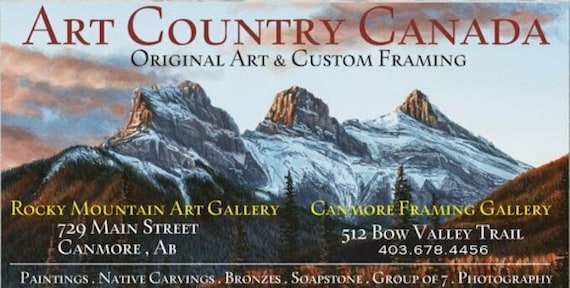This is a detailed business card for Art Country Canada, prominently featuring a color illustration of three snow-capped mountain peaks and a forest below in a landscape orientation. The card's design combines photographic representationalism with graphic design typography and includes a range of colors such as whites, browns, brownish red, yellows, blacks, and grays. 

At the top center of the card, bold serif dark red lettering states, "Art Country Canada," followed by smaller black text beneath it that reads, "Original Art and Custom Framing." Below the mountain illustration, there are two business locations featured. On the left, in yellow text, it reads "Rocky Mountain Art Gallery," and on the right, also in yellow text, it says "Canmore Framing Gallery." Both locations provide specific address information beneath their names: "729 Main Street, K-More, Alberta" for the Rocky Mountain Art Gallery and "512 Bow Valley Trail" for the Canmore Framing Gallery. 

Across the bottom of the business card, white text lists various artistic offerings: "Paintings. Native Carvings. Bronzes. Soapstone. Group of Seven. Photography." The entire design communicates the comprehensive artistic services and locations associated with Art Country Canada.